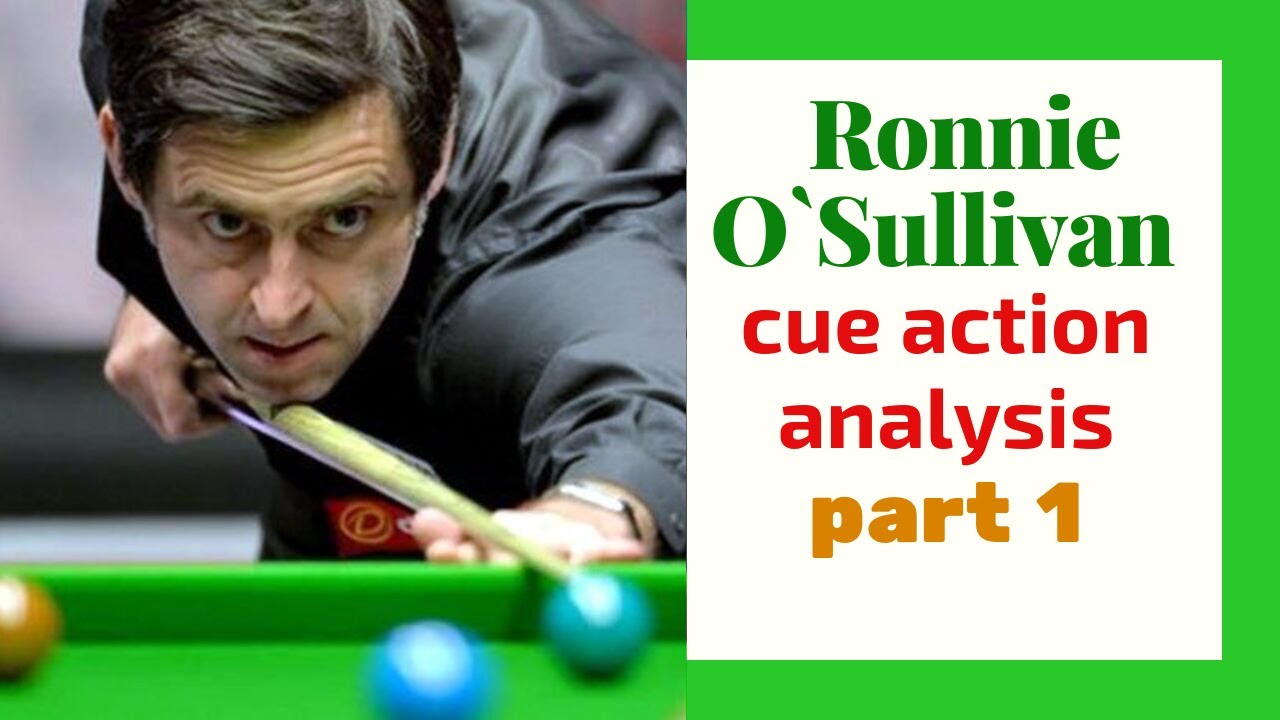The image appears to be a detailed cover of a book featuring the renowned professional pool player Ronnie O'Sullivan. The right side of the book cover is dominated by a white background with a green border. Prominently displayed in big green letters are the words "Ronnie" on the first line and "O'Sullivan" on the second line. Below this, in smaller red letters, it reads "Cue Action," followed by "Analysis" in similarly sized text. Finally, in bold golden-yellow letters, it says "Part 1."

The left half of the cover showcases a close-up image of Ronnie O'Sullivan. He is a middle-aged white man with deep wrinkles on his forehead, large eyes, and a slightly crooked nose. His lips are small, and he has dark brown or black hair. O'Sullivan is captured in an intense moment, bent over a bright green pool table, which matches the green of the border, preparing to take a shot. He is lining up the shot with precise focus, his chin almost resting on the cue stick. His left hand, palm up, is near the pool ball, with his right hand positioned further back. The table features three visible balls: an orange ball in the left corner, a blue ball in the center, and a teal-blue cue ball toward the right. O'Sullivan is dressed in a black suit or long-sleeve button-up shirt, adding to the intense, professional ambiance of the scene.